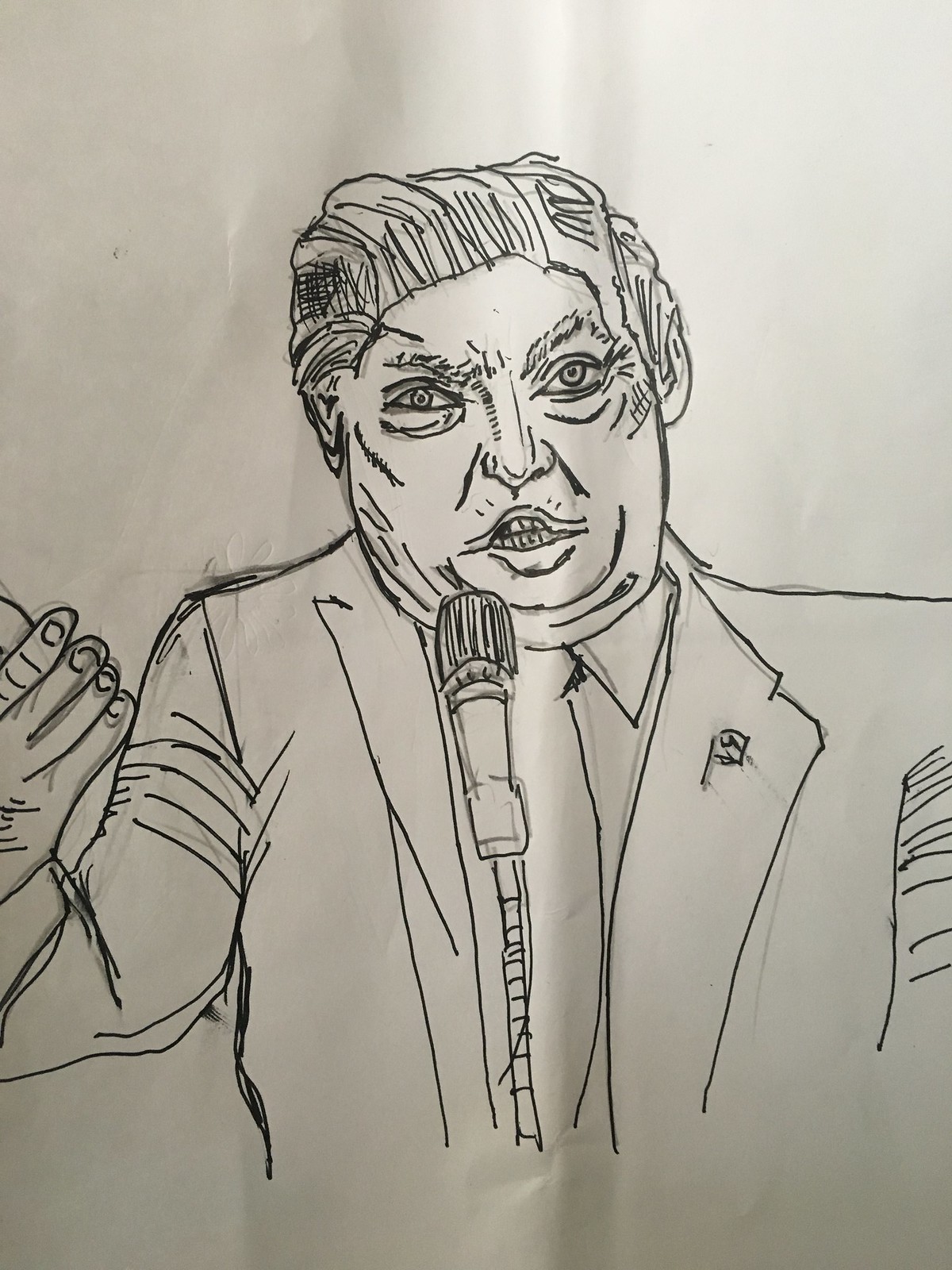This black and white photograph showcases a detailed drawing of Donald Trump, executed on a white sheet of paper that could be from a sketchbook, newsprint, or printer paper. The artwork appears to be rendered primarily in fine ink pen, with visible pencil lines hinting at initial sketches. The drawing captures Trump with his signature hairstyle, meticulously shaded to add depth. His expression is intense and somewhat angry, characterized by bulging eyes and a cruel, tightly curled mouth. Central to the image is a microphone, suggesting that he is speaking or addressing an audience. Adding to the realism, a small American flag pin adorns his lapel, complementing his typical suit and tie ensemble.